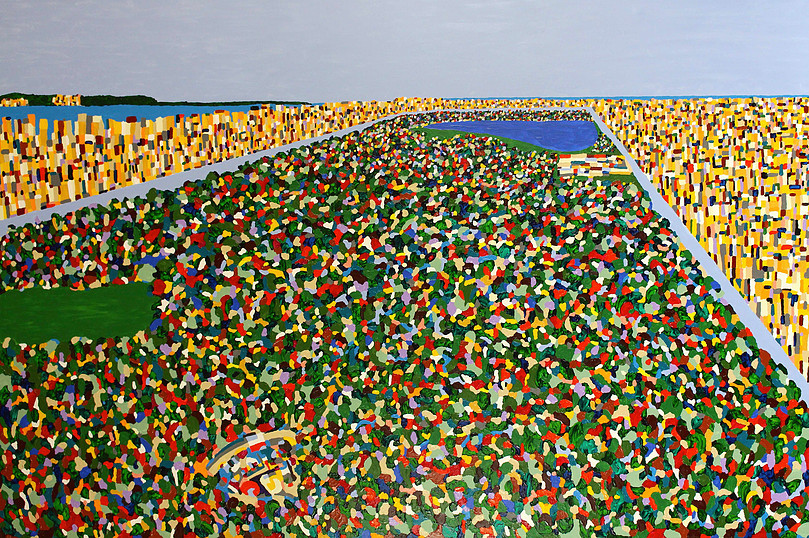This painting is a vibrant and abstract depiction of an outdoor setting, imbued with a multitude of colors and geometric shapes. Dominating the upper portion of the image is a blue skyline, creating a serene horizon. In the top left corner, mountainous forms create a rugged backdrop. Below the horizon, a band of assorted rectangular shapes in shades of brown, light brown, and orange suggests a cluster of buildings, which encircle a large, central, rectangular area reminiscent of iconic locations like the reflecting pool at the Washington Monument or Central Park.

The upper section of this central rectangle features a blue pond or small lake, adding a tranquil focal point. The remainder of this central space is filled with a mosaic of tiny, curved shapes in red, yellow, blue, and green, resembling a fragmented jigsaw puzzle. Intersecting the image are white or gray lines that span from left to right and along the back, creating divisions that hint at pathways or boundaries.

On the middle left side of the image, a small, green rectangular patch likely represents a grassy area. Throughout the image, bright colors such as red, green, blue, and yellow are prevalent, lending a lively and dynamic quality. These colors potentially symbolize people or vibrant city life within the abstract urban park scene. Flanking the image's colorful core, primarily yellow structures imply additional buildings. Lastly, the background showcases a vast, blue expanse, evocative of either an ocean or a large lake, culminating in a distant view of black mountains, hinting at further structures or natural features adorned with yellow highlights.